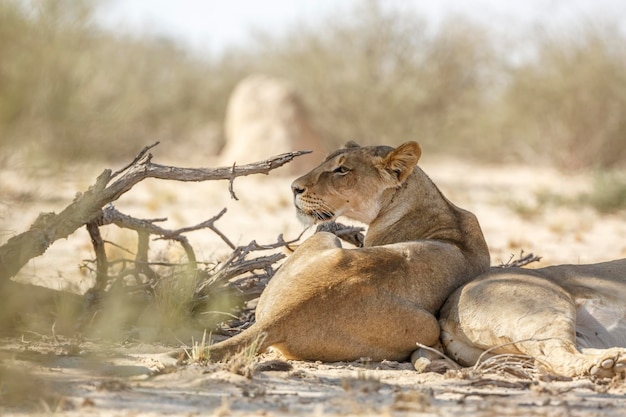In an evocative African desert setting, a female lioness lays partially in the shade, her tawny coat blending seamlessly with the sunbaked earth. She faces away from the camera, but her head is turned over her left shoulder, gazing intently to the viewer's left. Adjacent to her is a dried-out, scraggly tree branch, a testament to the arid environment. To her right, we glimpse the rear legs and part of the belly of another lion, likely another female, resting on its side. No cubs or male lions are visible. The background features scattered savannah scrub and a large, notable rock that appears to align with the tip of the lioness's nose. The shadows cast from left to right signal the sun's position, emphasizing the warmth and dryness of the day. Although there is a hint of green grasses among the arid scene, the overall impression is one of heat and tranquility in the wild.